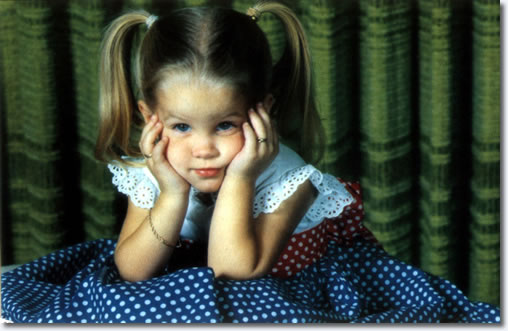The photograph features a young girl, estimated to be around five years old, posing in front of green, horizontally striped curtains that vary from medium to dark shades. She is a white girl with brunette hair styled in two ponytails, and she has blue eyes. Displaying a mock pouting or bored expression, she has her hands to her cheeks and elbows on her legs.

Her dress is particularly eye-catching; the top portion is white with lace and frills and has short sleeves adorned with crochet work. The middle section of the dress is red with white polka dots, while the skirt is blue, also dotted with white polka dots. She accessorizes with a bracelet and a ring, adding to her charming appearance.

The image has a professional feel, possibly retouched, evoking an old-fashioned aesthetic. Her pose suggests that the photo might be staged, perhaps for an advertisement or a formal portrait session.